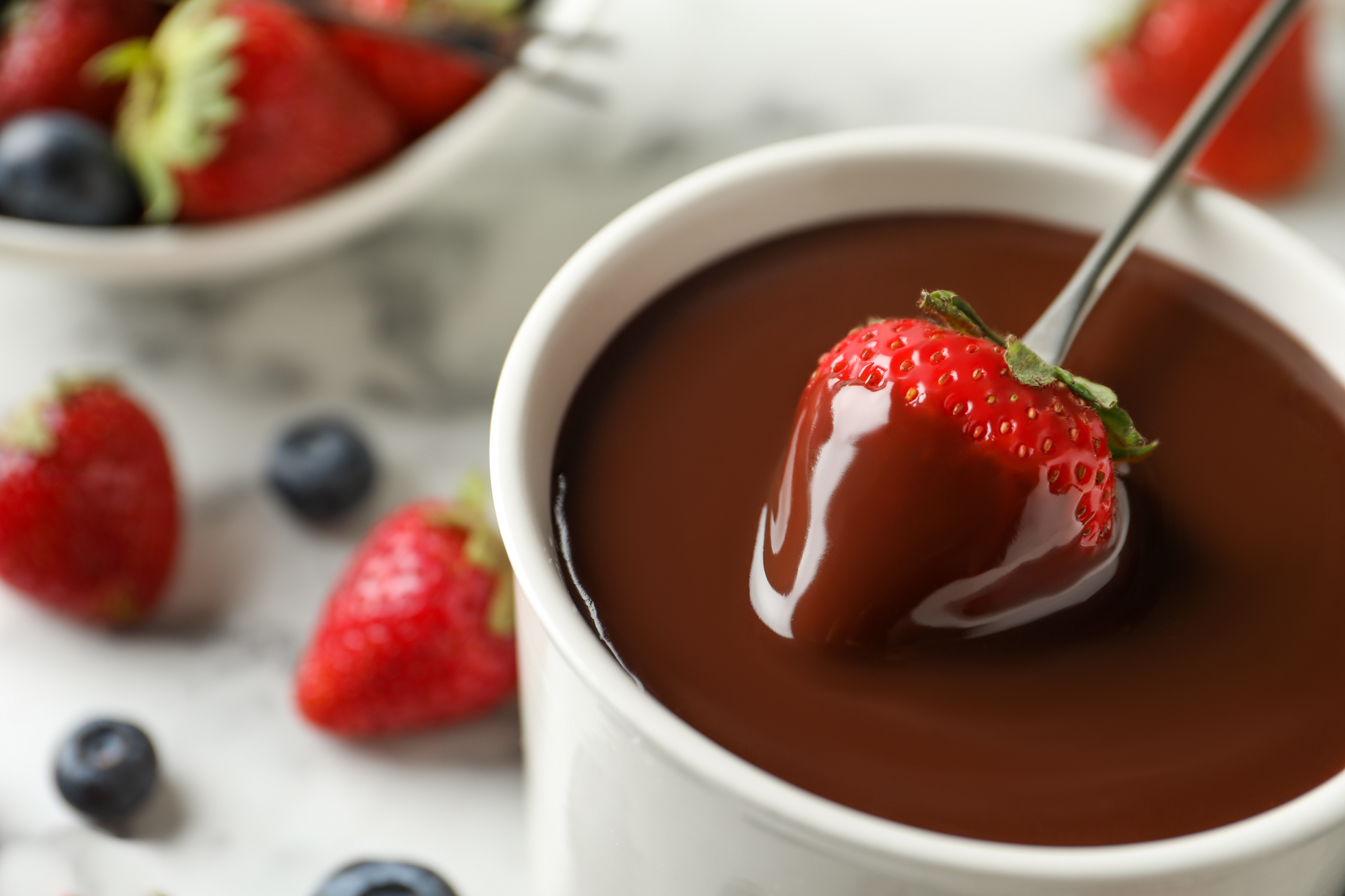In this vibrant and detailed image, the central focus is a bright red strawberry being dipped into a large white mug filled nearly to the brim with a rich, dark chocolate-like syrup. The strawberry, held delicately by a slim, metallic utensil that resembles a slotted flathead screwdriver rather than a spoon, retains its leafy green stem, adding to the visual appeal. As the strawberry is immersed, three-quarters of its surface glistens with the glossy syrup.

Surrounding the mug on a sleek, white marble-like counter are a few scattered whole strawberries and at least three blueberries, providing splashes of red and blue against the clean backdrop. To the left of the mug, a small white ceramic bowl brims with additional strawberries and blueberries, contributing to the abundance of fresh fruit in the scene. The overall composition captures the indulgence and vivid colors of the strawberries, the chocolate, and the assorted berries, creating a mouth-watering visual experience.